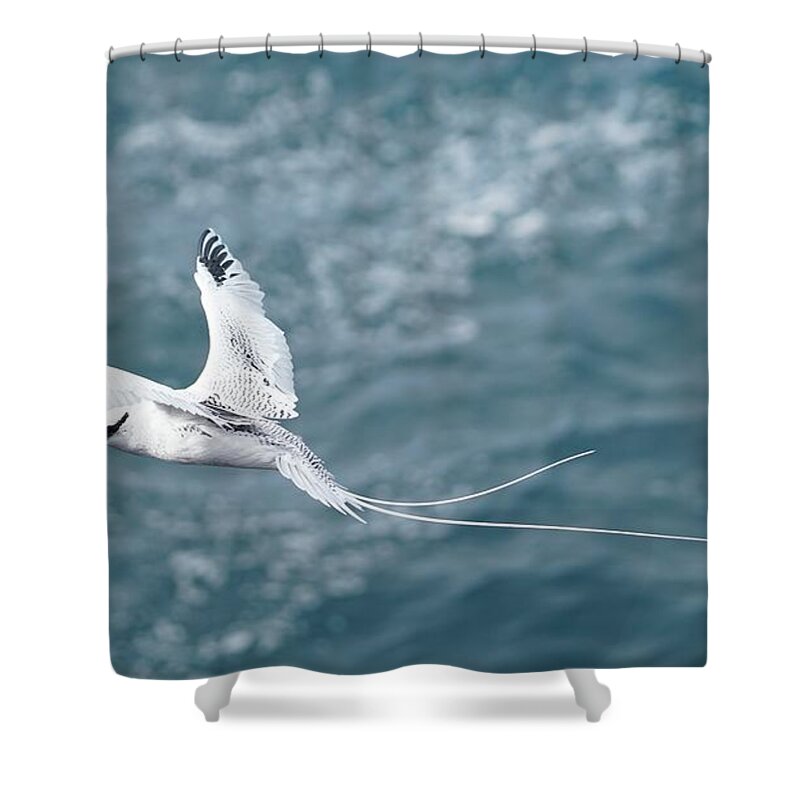The image showcases a highly decorative fabric shower curtain suspended from a white shower rod, which extends horizontally across the top. Black shower curtain rings are evenly spaced along the rod, securing the curtain. The curtain features a vivid photograph of a tern, a type of bird, in mid-flight, gliding towards the left. The bird's head is not visible; instead, we see its predominantly white body with a distinctive black stripe near its neck. Its outstretched white wings are tipped with black feathers, and two long tail feathers extend in a V shape. The background behind the bird is a bluish blur, suggesting water ripples, adding to the overall serene and natural ambiance of the image. At the bottom of the curtain, two grayish bathtub legs are visible, indicating the presence of a bathtub.